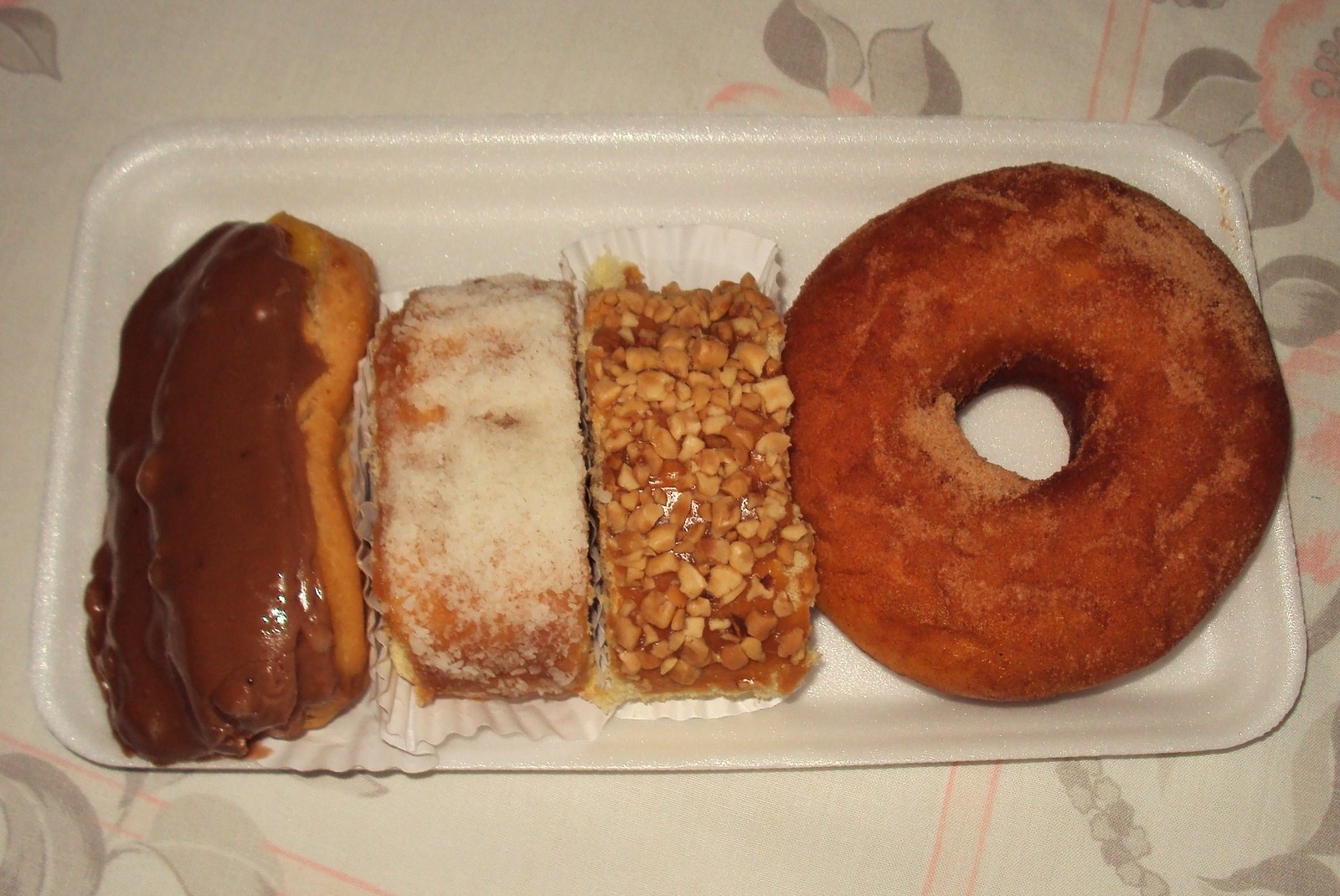This color photo features a selection of diverse pastries carefully arranged on a white rectangular styrofoam plate, which is set on a white tablecloth adorned with a faded pink and gray floral design, giving it a vintage feel. On the left side of the tray, there is a chocolate-coated eclair. Beside it, in the center, lies an oblong slice of yellow cake nestled in a cupcake wrapper, topped with white sugar frosting. Next to this, towards the center-right, appears to be another oblong cake slice, also in a cupcake wrapper, generously covered with crushed nuts and possibly a sticky toffee glaze. Finally, on the far right, there is a large donut heavily dusted with cinnamon sugar, its darker hue suggesting it might be slightly overcooked.